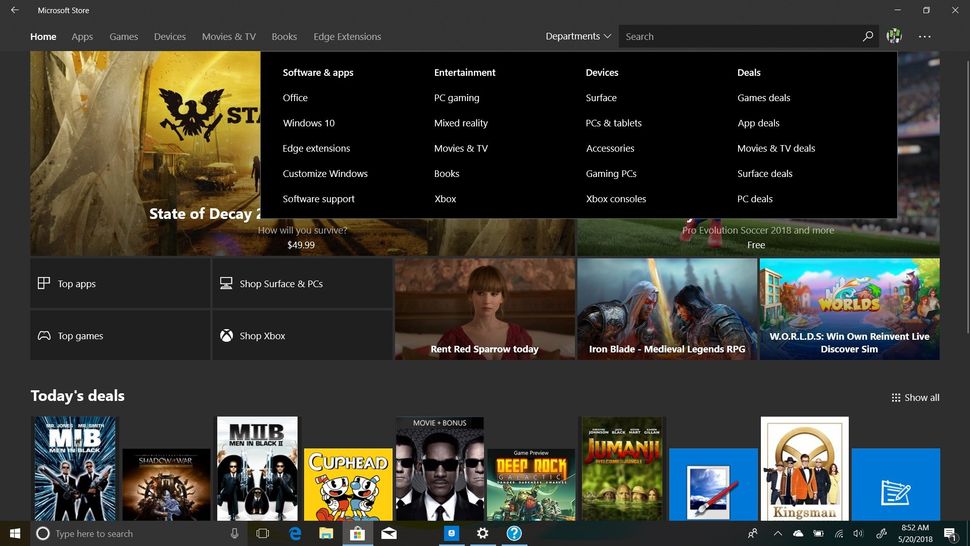The image depicts the interface of the Microsoft Store. In the top-left corner, "Microsoft Store" is prominently displayed in white text. Directly below, a series of navigation tabs are organized with "Home" highlighted in white, and adjacent tabs in gray, including "Apps," "Games," "Devices," "Movies & TV," "Books," and "Edge Extensions." On the right side of these tabs, there's a "Departments" dropdown menu indicated by a downward arrow and a darker search box.

Beneath the navigation tabs, various categories are listed as subtitles. On the left, it reads "Software and Apps," followed by subcategories such as "Office," "Windows 10," "Edge Extensions," "Customize Windows," and "Software Support." Adjacent to that, under "Entertainment," subcategories include "PC Gaming," "Mixed Reality," "Movies & TV," "Books," and "Xbox."

In the next column titled "Devices," the subcategories are "Surface PCs & Tablets," "Accessories," "Gaming PCs," and "Xbox Consoles." Following this, under "Deals," the subcategories include "Game Deals," "App Deals," "Movies & TV Deals," "Surface Deals," and "PC Deals."

The main visual content area features multiple images representing different games and movies. Titles such as "State of Decay," "Iron Blade," and terms like "Our Worlds," "Win," "Own," "Reinvent," "Live," and "Discover" are displayed prominently. 

At the bottom, a section labeled "Today's Deals" showcases movie and game titles such as "MIB Men in Black," "Shadow of War," "Cuphead," "Deep Rock Galactic," "Jumanji," and "Kingsman." Additionally, the Windows taskbar is visible at the very bottom of the interface, providing a familiar touch of the Windows UI.